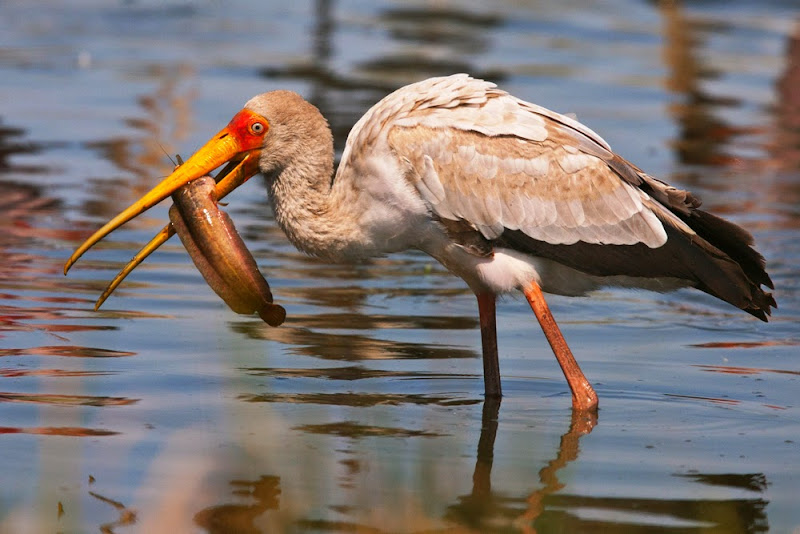In this image, a yellow-billed stork stands in the shallow waters of a marsh, facing left. The stork has a striking long yellow beak, with a hint of orange around its sharp red eyes. Its legs are long and pink, extending down to the bottom of the water, highlighting the shallowness of the setting. The bird's plumage is a mix of light brown, white, and dark brown feathers, with distinct black feathers under its tail and white feathers near the top of its legs. In its beak, the stork holds a brown sea creature with long fins and a small tail, possibly a shrimp, given the visible antennas. The scene is well-lit, suggesting it is midday, and the stork's reflection can be seen in the tranquil water, adding depth to the image. The bird is positioned slightly off-center to the right, with the captured sea creature extending towards the left.